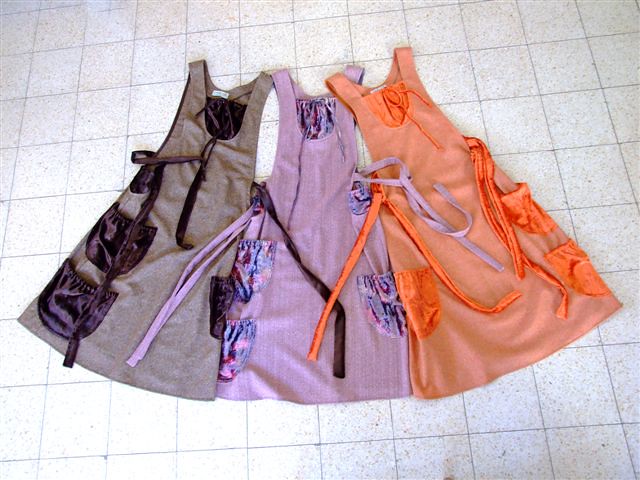This photograph, taken in color with a clear vantage point from a standing position, captures the scene of a kitchen's speckled linoleum floor with medium-sized square tiles featuring beige, white, and brown variegations and visible gray mortar lines. The focus of the image is on three identical sundresses, laid out side by side. Each dress features spaghetti straps, multiple pockets, and a sash that can be tied. The dress on the left is a light brown with dark brown velvety pockets and a sash, darker brown accents in the bodice area, and a scoop neck not too deep. The middle dress is lavender with floral patterned pockets in purple, pink, and blue, and a matching purple sash. The dress on the right is orange with darker orange pockets, bodice, and sash. Each dress has a gathered bodice and is laid out straight, central in the frame.